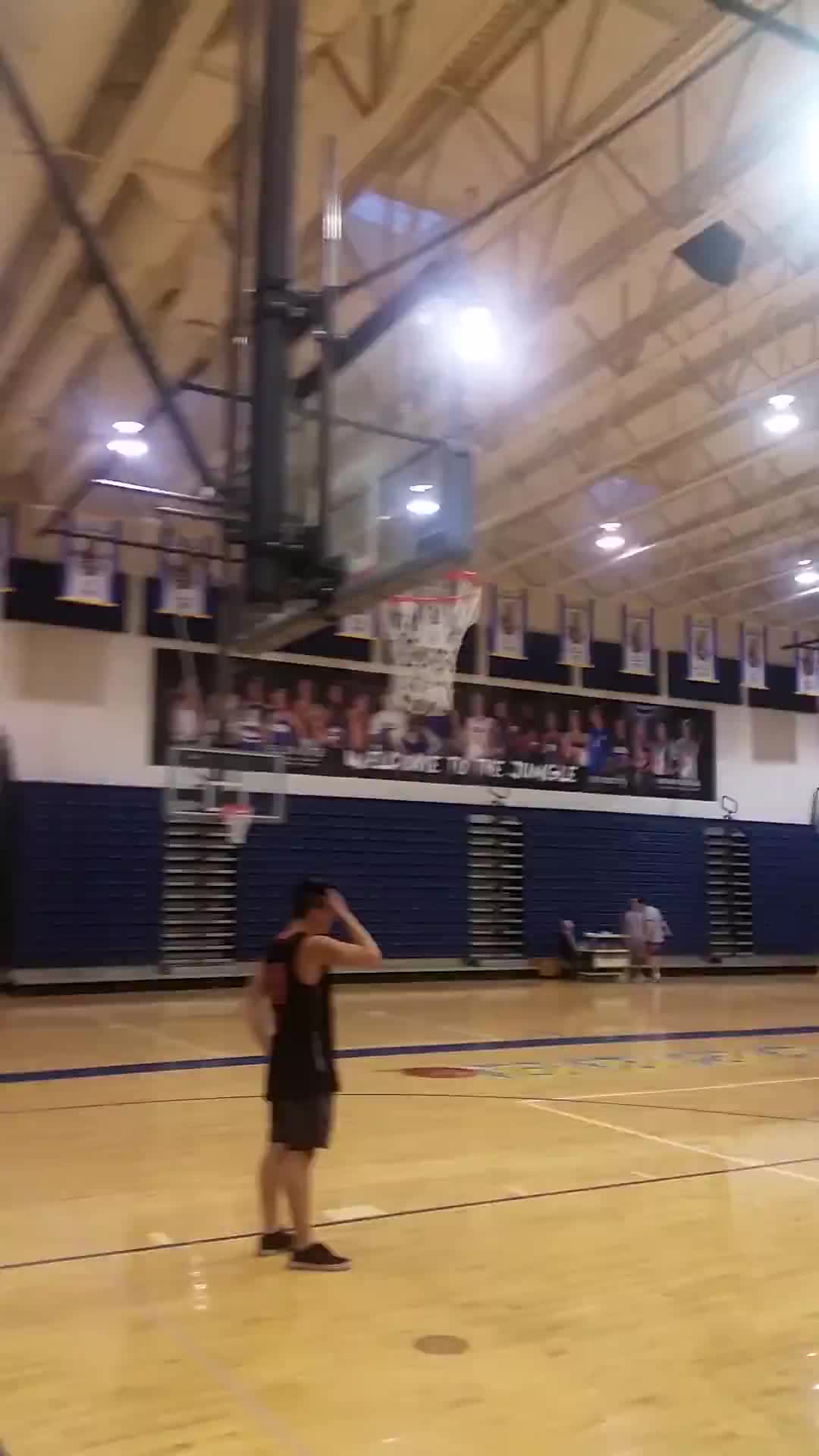The photograph captures a scene inside a large, well-lit gymnasium with high ceilings, featuring a basketball hoop prominently in the foreground. A young male player, dressed in a black tank top, black shorts, and black shoes, stands beneath the basketball hoop. He has dark hair, and his right hand is scratching his head while his left hand rests on his hip. The glossy pine floor of the court, marked with game lines, lies beneath his feet. 

In the background, the blue bleachers are folded, and there appears to be minimal activity, suggesting this may be a practice session rather than an actual game. Further back, another individual stands near a table positioned against the opposite wall. Above them, a large banner stretches across, adorned with images of players and the bold slogan "Welcome to the jungle." This banner is flanked by several championship banners hanging above it. Light fixtures and possibly a skylight illuminate the entire gymnasium, adding to the bright indoor setting.